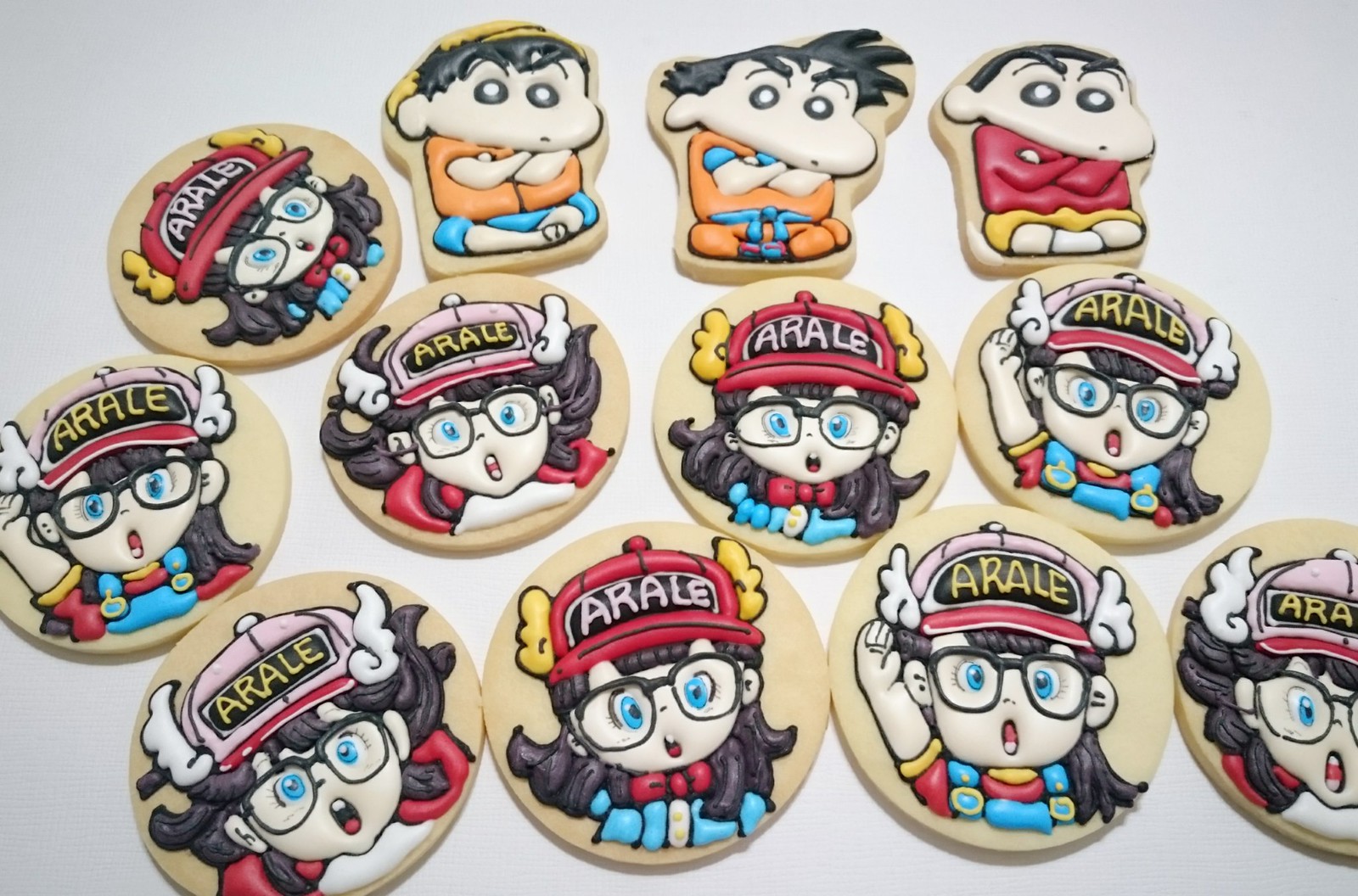The image features a collection of round, elaborately decorated items that appear to be cookies, possibly toys, stamps, or magnets. They are arranged roughly in three rows of four against a light gray or white background, though the rows aren't perfectly neat. The majority of these items depict a cartoon figure of a girl with blue eyes, glasses, and long black or dark gray hair, wearing a cap that prominently features the word "A-RALE" on the front. Her cap has wings on the sides, varying in color from white to yellow. She is shown with an open mouth as if yelling, and is dressed in a blue denim dungaree with a white top underneath. The cap comes in different colors, including red and pink. In contrast, the top row features three images of a boy with black hair, shown sitting cross-legged with his hands clasped. The boy's appearance varies slightly: he wears an orange hat in one, appears with messy hair in another while seated in a dojo, and lastly, he is shown in a white hoodie and black pants with neatly combed hair. Both characters are depicted with distinctive, expressive cartoon features, making the entire collection vibrant and detailed.